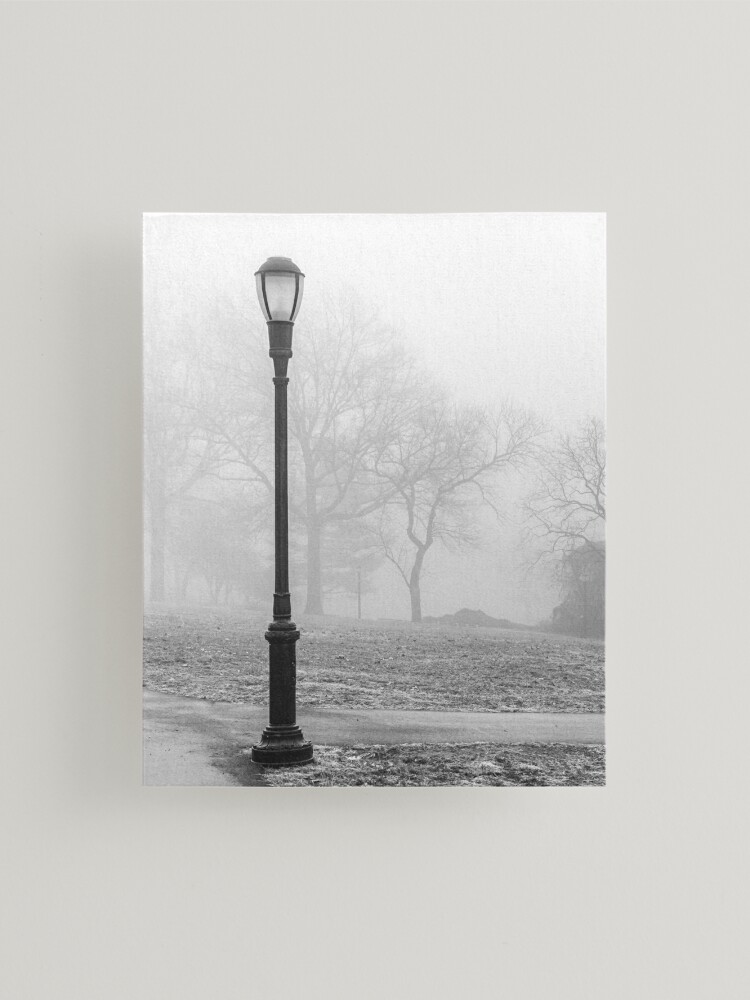This striking black-and-white photograph captures an ornate streetlight positioned near the intersection of two small paved paths, creating an L-shaped corner at the bottom left of the image. The streetlight, prominently placed in the middle left side of the picture, boasts a cylindrical base that narrows into a slender black pole. Its top features a glass globe encased in a decorative black cap with intricate molding details. The setting appears to be a park, with a small open field and several low bushes framing the scene. The background is filled with the silhouettes of dark-colored leafless trees, their tall, spindly branches stretching into a foggy, light gray sky, hinting at winter. Scattered patches of what looks like lingering snow rest on the barren ground and mingle with the dry grass, enhancing the wintry ambiance.